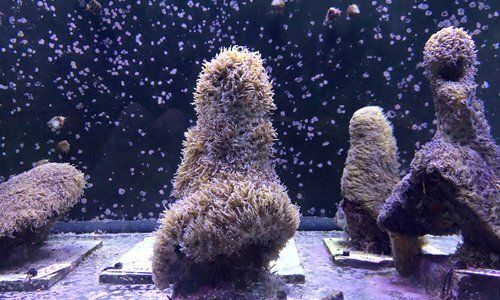The image depicts a surreal and intricate underwater scene, possibly captured inside an aquarium or in the deep sea. The photograph showcases a black or deep blue backdrop speckled with numerous pale, whitish, and light purple dots, reminiscent of marine life like shrimp or air bubbles gently drifting through the water. In the foreground, there are four fuzzy, statue-like figures that evoke anemones, corals, or some type of algae. These figures are mounted on square, metal panels with screws, hinting at an artificial setup such as an aquarium installation or a sunken ship's deck reclaimed by marine wildlife. Each anemone-like structure is unique in shape and color, ranging from light brown and yellowish hues to a mix of green and dark yellow leaves. The fuzzy textures and undulating forms suggest movement, possibly swaying with underwater currents. Small sensors or water measurement devices attached to each panel underline the scene’s possibly experimental or observational nature. Amidst this eerie and captivating setup, small fishes swim by, adding life to the otherwise tranquil and mysterious tableau.